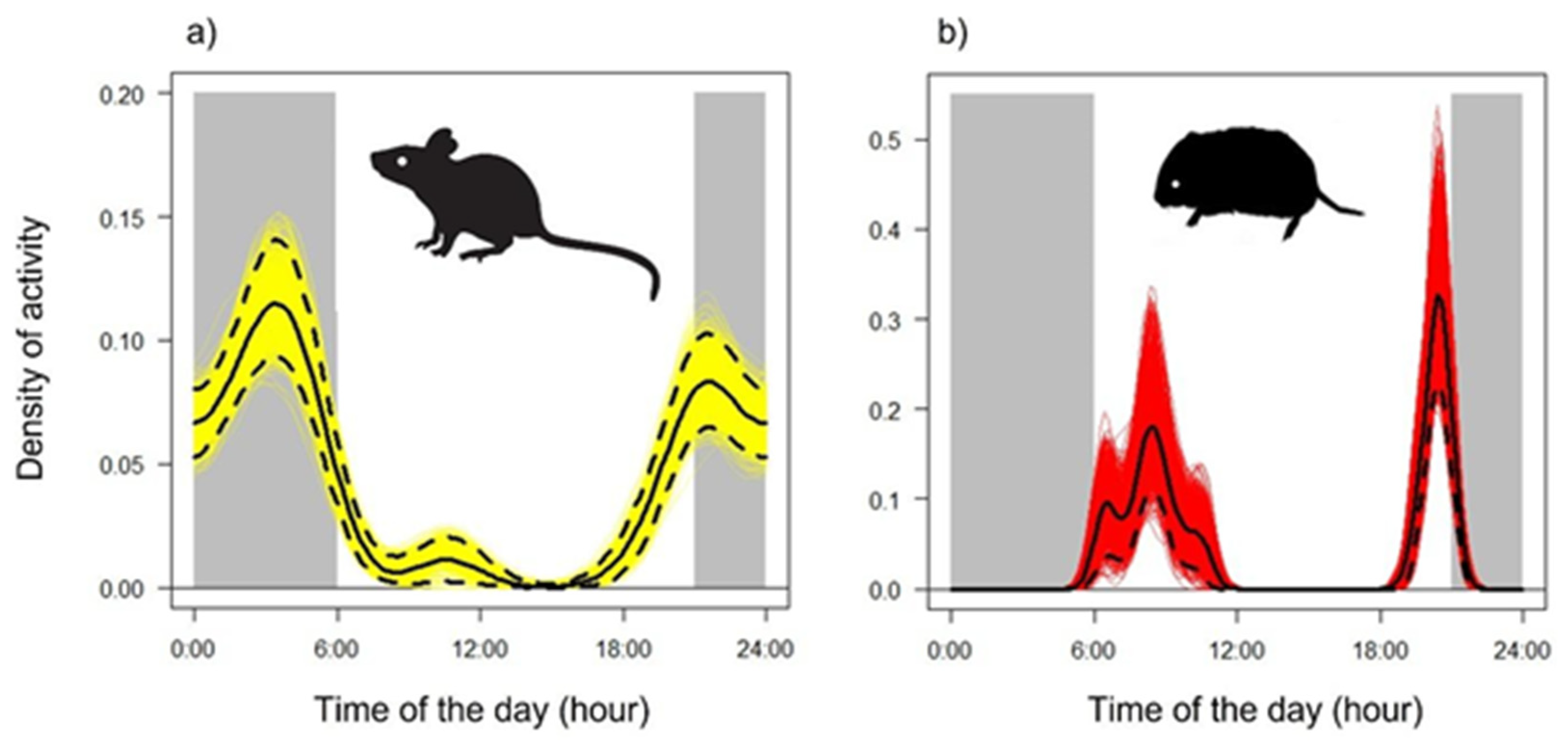The image consists of two distinct charts, labeled A and B, providing an infograph about the activity patterns of a mouse and a hamster. In the left chart (A), there is a shadow image of a mouse. The Y-axis, labeled "Density of Activity," runs vertically, while the X-axis at the bottom indicates "Time of Day" in hours. The mouse shows varying levels of activity throughout the day, with peak activity around 3 AM and noticeably lower activity during midday. 

In the right chart (B), a shadow image of a hamster is featured. Similar to chart A, its Y-axis is labeled "Density of Activity," and the X-axis marks the "Time of Day" in hours. The hamster displays sporadic activity patterns, with significant peaks of activity around 8 PM and early in the morning, but periods of inactivity scattered throughout the day.

Overall, the infograph effectively compares the more consistent, though slightly lower, daily activity of the mouse with the more sporadic and distinct activity peaks of the hamster.